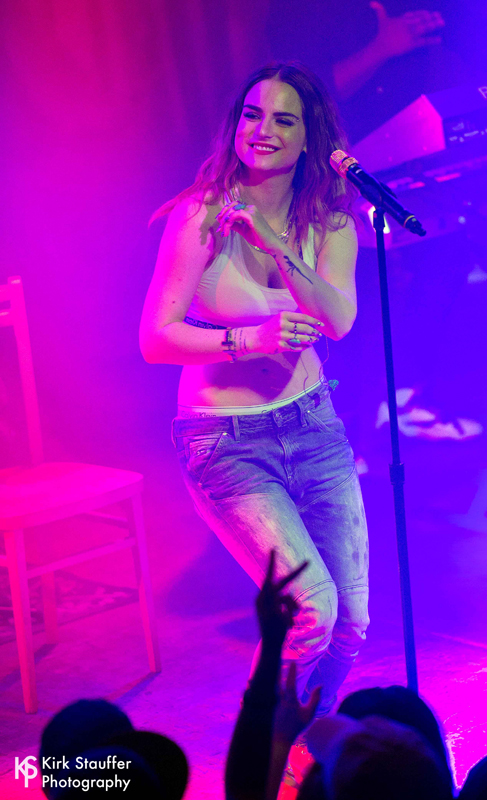This photograph captures a dynamic concert scene dominated by pink and blue lighting, with the hues blending across the image. In the lower left corner, the text "Kirk Stouffer Photography" is written in white, with a distinctive "KS" logo beside it. The background showcases a gradient from pink on the upper left, transitioning to blue on the upper right, with a mix of both colors filling the lower parts of the image. 

At the center, a young woman, resembling the singer Jojo from the early 2000s, stands on stage. She is a Caucasian woman in her late teens to late 20s, with shoulder-length, slightly wavy brown hair, and she appears to be wearing subtle makeup. She is dressed in a white tank top and denim jeans, her casual yet stylish attire fitting the concert atmosphere.

She stands in front of a microphone on a stand, singing to an unseen audience. The top of the microphone is a lighter color, while the handle is black. Behind her, to the right, a chair under pink lighting adds depth to the scene, casting a shadow to the left. To the far right of the image, a DJ or another musician can be seen, faintly illuminated by the stage lights.

The lower portion of the image hints at the presence of the crowd, with various silhouettes including hands showing gestures like the peace sign. The vibrant environment and lighting, combined with the performer and the audience, encapsulate the energy and excitement of a live concert.